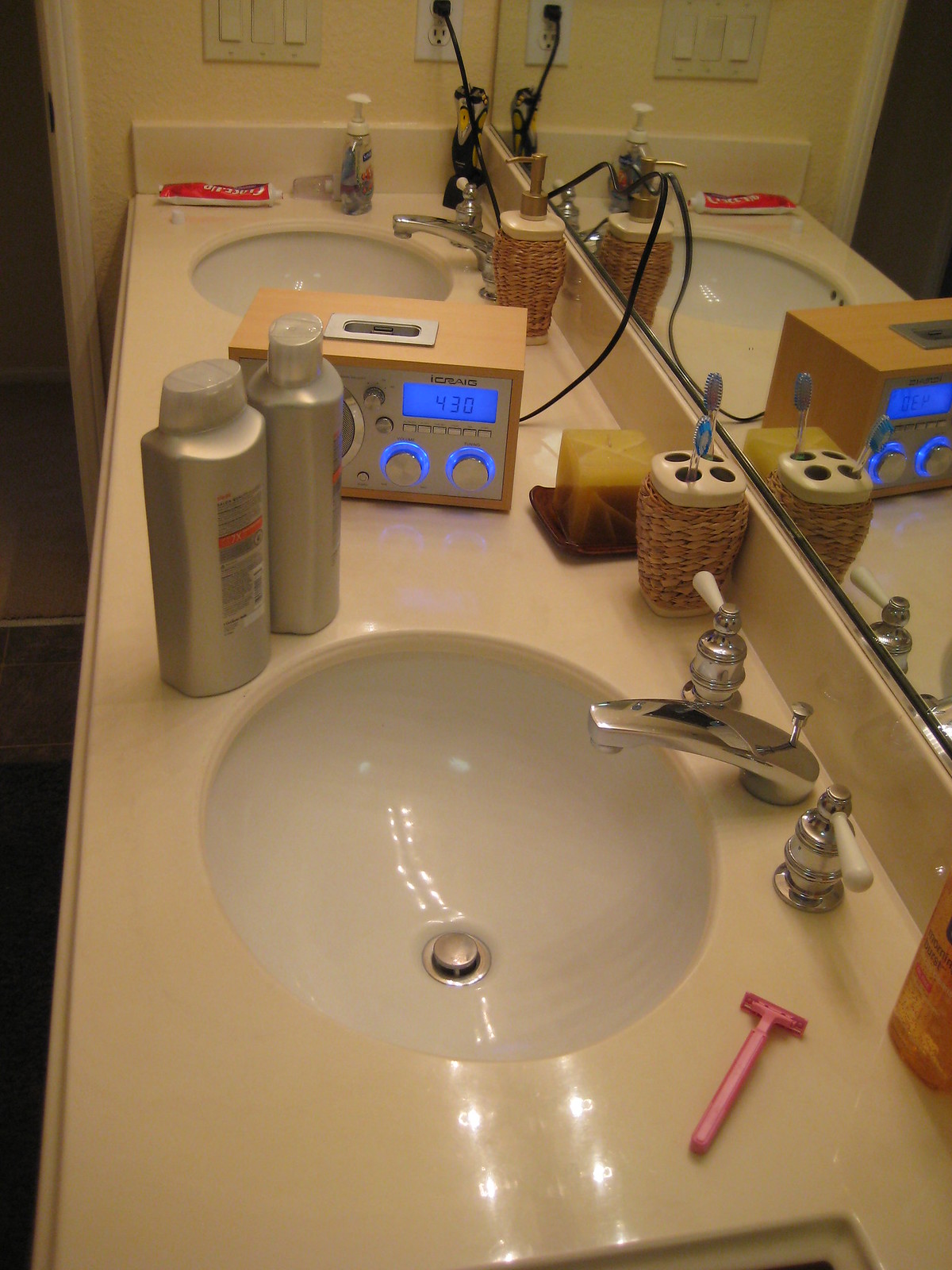The photograph captures a rectangular-shaped bathroom countertop and sink set, viewed from an angle that showcases the right side of the counter. Dominating the top right section of the image is a large mirror that spans the entire length of the wall behind the backsplash, reflecting all objects on the counter and an opened, white painted doorframe located in the top left corner.

The tan-colored countertop features two recessed white sink basins, each accompanied by a slightly curved, rectangular-shaped stainless steel faucet. Embedded within the countertop, near each sink, are two white-handled controls for managing the water flow. Centrally positioned between the sinks is a brown radio, which is plugged into an outlet via a black cable. The radio boasts a silver faceplate adorned with multiple knobs, a built-in speaker, and a blue LED screen, adding a touch of modernity to the bathroom's design.